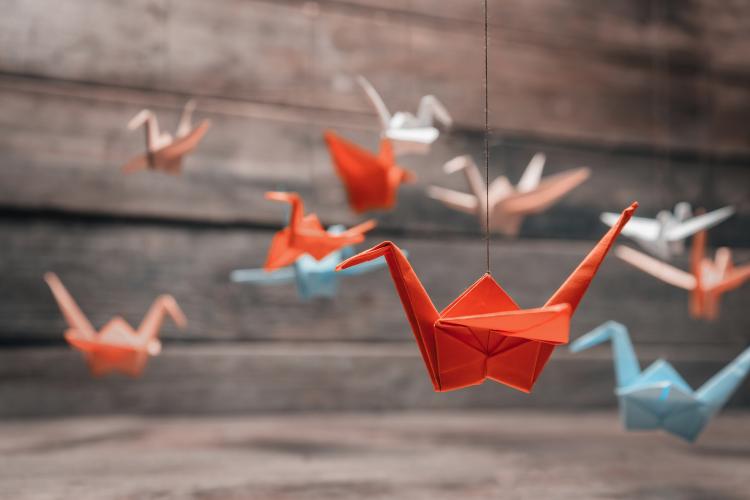This photograph features approximately 10 origami cranes, all suspended from strings against a backdrop of horizontal wooden slats. The central focus is a sharp, reddish-orange crane situated slightly right of center and facing left. This crane is distinct and has a black string attached to it, leading upwards out of the frame. Positioned to its bottom right is a blue crane, also facing left but slightly blurred. Above and around these primary cranes are several more, including a white crane and a red crane, all with varying degrees of blur. These additional cranes are predominantly in shades of red, pink, and white. The wooden slats in the background are horizontal and range in color from tan and brown towards the top to a darker gray near the bottom, giving the setting a rustic, aged appearance.